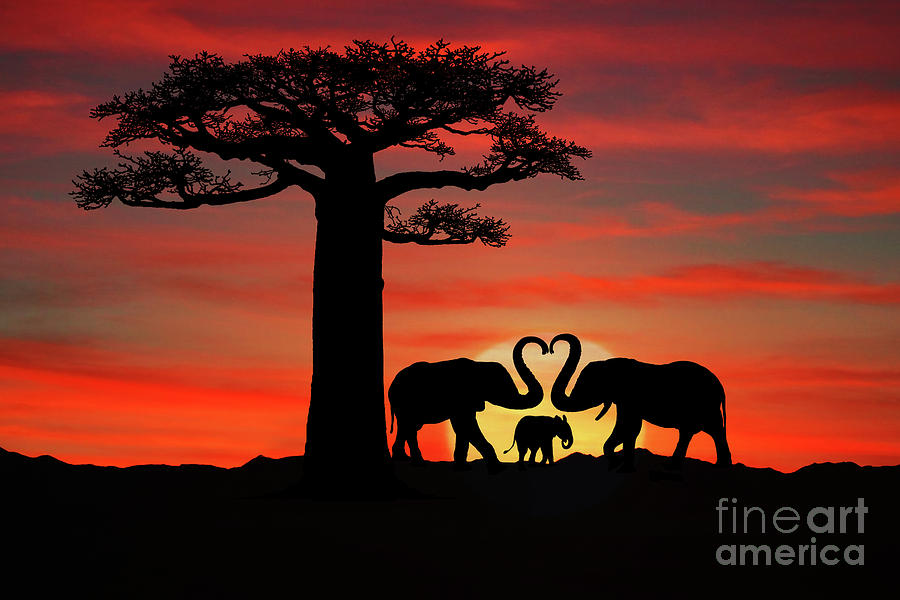The image is a digital or computer-generated artwork depicting a picturesque sunset over a savanna-like landscape. The backdrop features a sky painted in brilliant hues of blue, pink, red, and orange, fading into a rich, warm glow as the sun sets near the bottom center of the composition. Silhouetted against this vibrant sunset, a large tree occupies the left third of the image, characterized by a tall, sturdy trunk and leafy branches that spread out only at the top. 

To the right of the tree, the foreground is adorned with the black silhouettes of two adult elephants facing each other, their trunks raised and intertwined to form a heart shape above their heads. Nestled between them stands a baby elephant, also in silhouette, centered perfectly in the space beneath the heart formed by the adult elephants' trunks. The textured, uneven ground beneath them is also rendered in black, enhancing the silhouette effect. In the bottom right corner, the image is overlaid with the text "Fine Art America," indicating its artistic source. This scene, captured in shadow and color, conveys a serene and heartwarming moment at dusk.